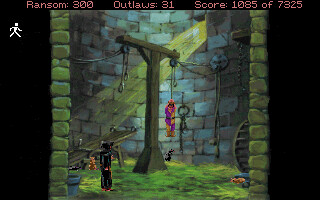This color screenshot is taken from the video game "Conquest of the Longbow." The top of the image displays game statistics with text reading "Ransom 300, Outlaws 31, Score 1085 of 7325" from left to right. At the center, the scene is framed by imposing stone columns on either side, creating a dramatic circular focal point. Dominating the right side, a device similar to gallows suspends a figure clad in purple and yellow from chains, leaving them hanging off the ground. Beneath this, a shadowy figure dressed entirely in black with a hood stands ominously. A single window breaks the surrounding stone architecture at the top, allowing a beam of sunlight to stream diagonally from the top right to the bottom left corner, illuminating the green grass or hay strewn across the ground. The overall composition creates a tense and immersive atmosphere within the game.